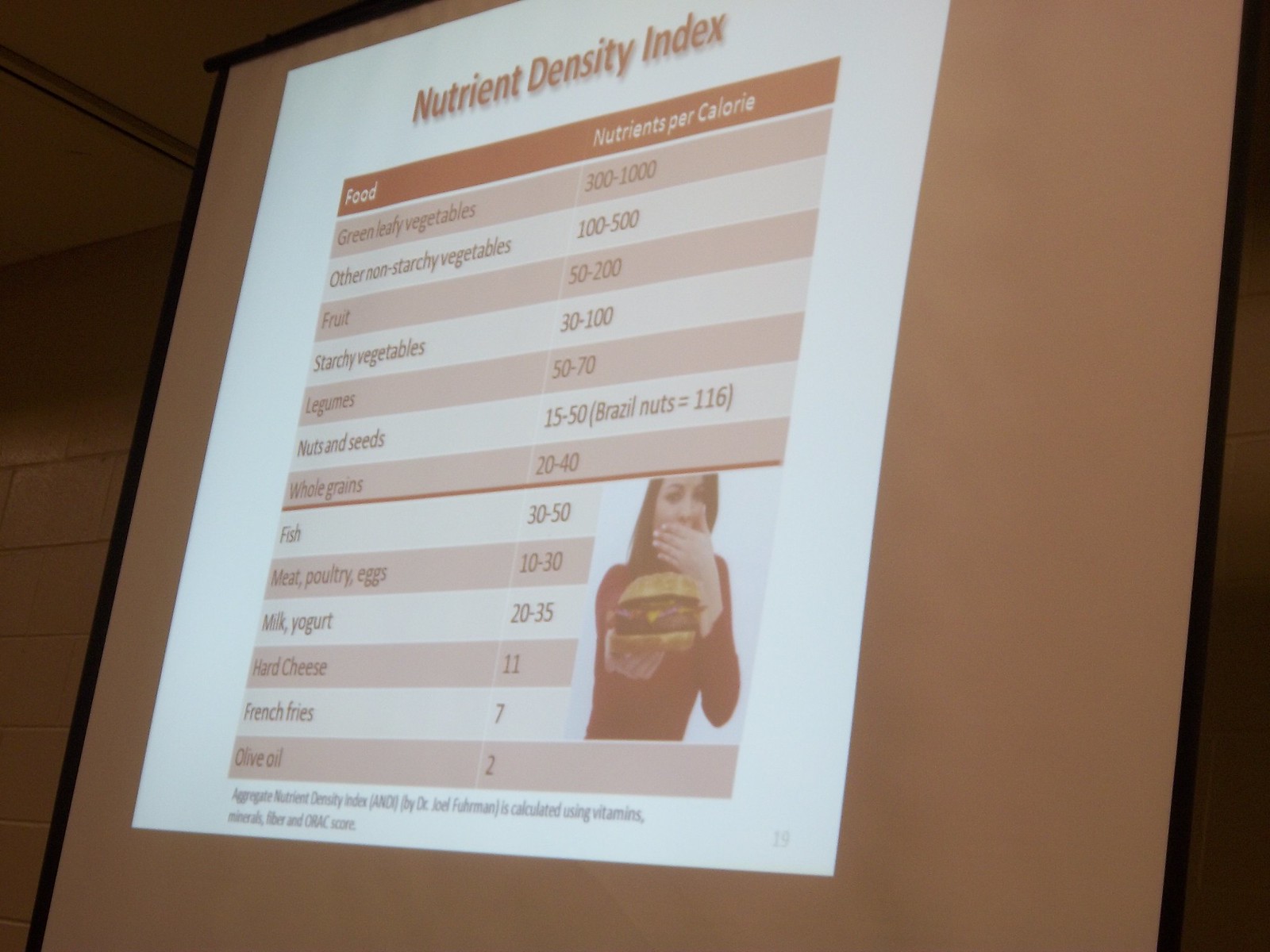This is a detailed photograph of a presentation slide being projected onto a pull-down screen, which is slightly tilted, making the right side closer to the viewer than the left. The ambient lighting and projection give the image an overall brown and orange tint. The screen is bordered in black and positioned against a background featuring a bit of ceiling and a wall, which has wooden molding.

The title of the chart on the screen reads "Nutrient Density Index," which measures nutrients per calorie for various foods. The chart has two main columns: the left column lists different types of food, while the right column details the nutrient density per calorie. The rows alternate in color between light red and white for better readability.

Listed under the food category are: green leafy vegetables, other non-starchy vegetables, fruit, starchy vegetables, legumes, nuts and seeds, whole grains, fish, meat, milk, yogurt, hard cheese, French fries, and olive oil. Notably, green leafy vegetables and other non-starchy vegetables are highlighted as having significantly higher nutrient density compared to fish and meat.

In the lower right-hand corner of the chart, there is a photograph of a woman holding a cheeseburger with her right hand, partially covering her mouth with her left hand, adding a visual element to the presentation.